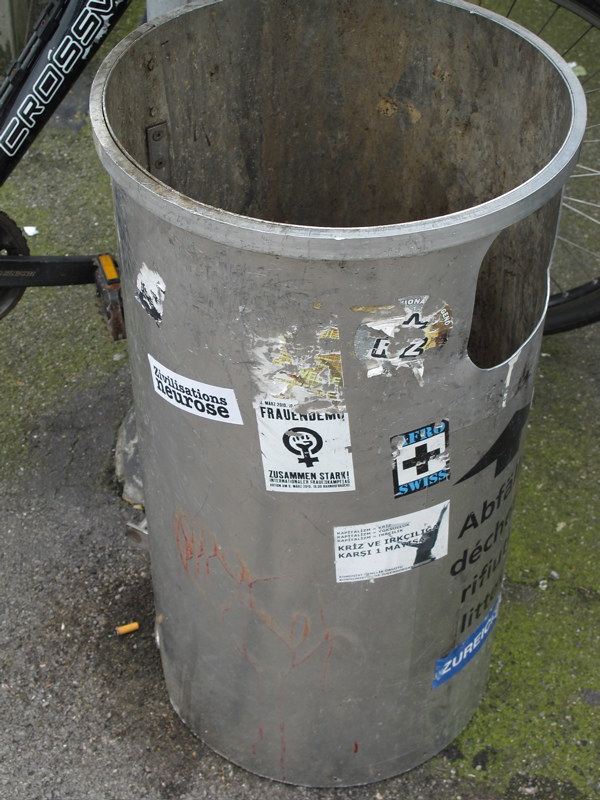A close-up image showcases a tall, tube-shaped plastic trash can, predominantly gray and heavily discolored with yellow water marks and dirt inside. The exterior of the trash can is adorned with a variety of stickers, many of which have been torn or peeled off, revealing layers of neglect. The remnants of black, white, and some blue stickers are visible, adding to the ragged appearance. The trash can has a side hole on the top right for inserting garbage, suggesting it may have once had a lid which is now missing. It appears bolted to a pole, standing on an asphalt ground that is dirty and speckled with green moss-like growth. A cigarette butt lies discarded on the ground to the left of the trash can. In the background, a black bicycle is partially visible, displaying the crossbar, pedal, chain ring, and the thin front tire with spokes, adding to the cluttered and worn-down setting.